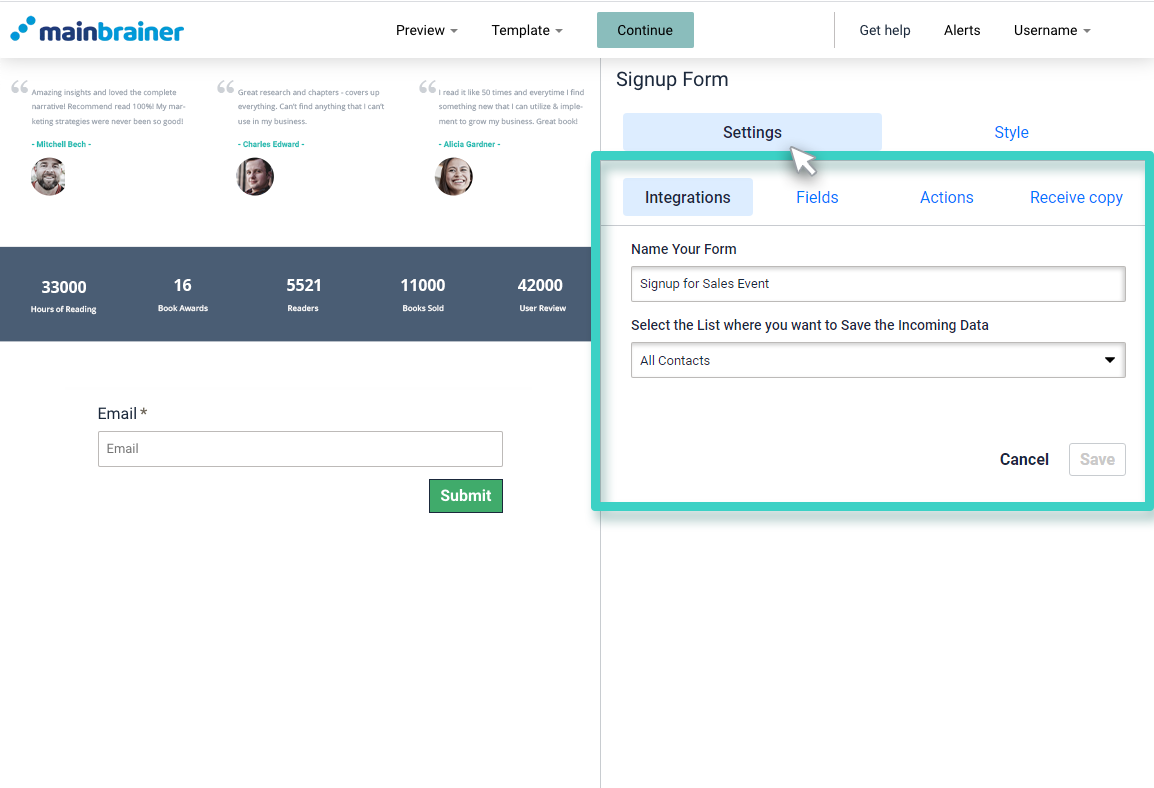The image appears to be a screenshot from a website called Mainbrainer, identified by the blue "Mainbrainer" logo in the upper left corner. The user has clicked on the "Continue" button, which is illuminated in green. A pop-up box with a green border and a white interior has appeared on the screen.

Within the pop-up box, it indicates that the user has navigated to the "Integrations" section. The instructions in the box prompt the user to name their form and sign up for the sales event, and to select the list where they want to save the incoming data, with an example option named "All Contacts." The bottom right corner of the pop-up contains a dark, prominent "Cancel" button and a less visible "Save" button. Above the pop-up, the word "Settings" is bolded, suggesting that this section has been accessed, and a white arrow points to the bolded "Settings," indicating recent interaction.

On the left side of the image, testimonials from users of Mainbrainer are displayed. There are three pictures featuring two men and one woman. The first testimonial is from Michael Beck, a white man with a beard, who states, "Amazing insights and love the complete narrative. My marketing strategies have never been so good." These testimonials are meant to promote and endorse the Mainbrainer platform.